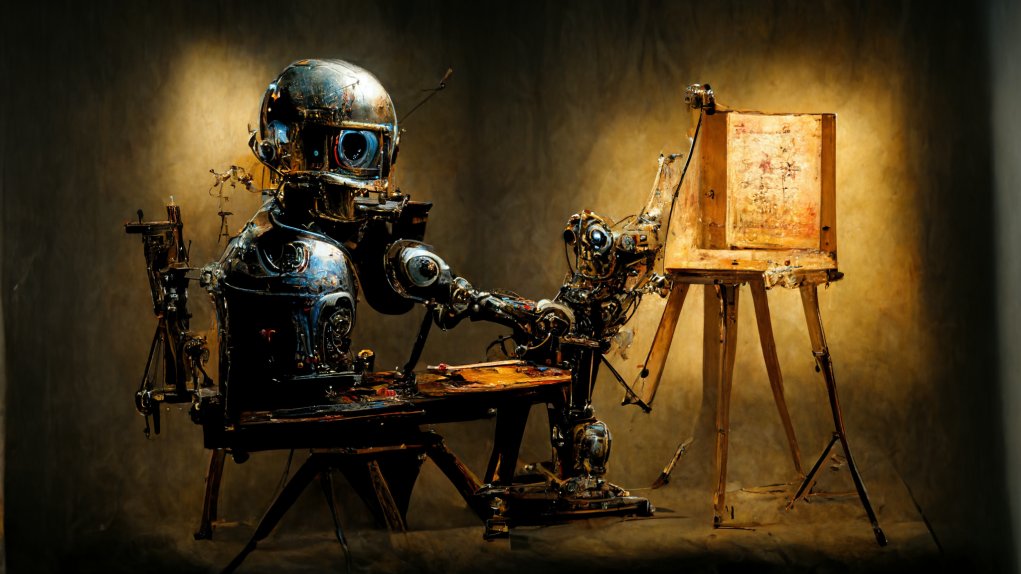This rectangular image, approximately 6 inches wide by 3 inches high, appears to be a detailed digital art piece with darkened edges and corners, giving way to a lighter interior that highlights the setting of an old, dilapidated building with grey or dark walls. The focus is on a wooden easel, partly held up by a mechanical, humanoid robot that appears broken and damaged. The robot, with a round head, robotic arms, and a cylindrical torso, sits on the floor. Its body is complex with wires hanging out and multiple limbs, including one arm extending towards the easel. The easel itself is in disrepair, featuring broken legs, some reattached with bits of metal. Scattered around are canvases and paint, with noticeable paint spewing about, suggesting an intense, almost chaotic painting ambiance. The robot seems to be engaging with the easel, creating an intriguing mix of mechanical and artistic elements amidst the antiquated setting.